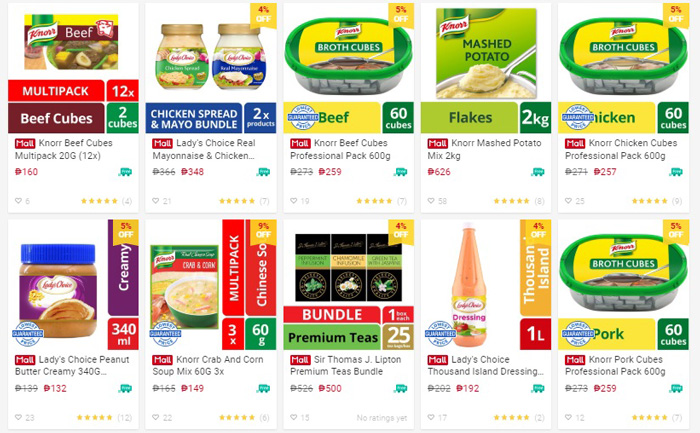This image is a screenshot of a shopping website displaying various products available for sale, complete with photos and prices. The layout is divided into two sections, each showcasing 5 products, making a total of 10 products.

In the top-left corner of the image, there is a listing for "Knorr Beef Cubes Multipack 20 grams 12X," priced at $1.60. The product details include a star rating and additional information that it is a multipack containing 12 units, with each unit comprising 2 cubes.

Moving to the right, the next listing features "Ladies Choice Real Mayonnaise and Chicken." To its right is "Knorr Beef Cubes Professional Pack 600 grams." Further right is "Knorr Mashed Potato Mix 2 kilograms," and finally, in the top-right corner, "Knorr Chicken Cubes Professional Pack 600 grams."

The bottom row starts with "Ladies Choice Peanut Butter Creamy 340 grams." Next to it is "Knorr Crab and Corn Soup Mix 60 grams 3X." Following this is "Sir Thomas J. Lipton Premium Teas Bundle." To the right of it is "Ladies Choice Thousand Island Dressing," and the final product in the bottom-right corner is "Knorr Pork Cubes Professional Pack 600 grams 60 cubes."

Each product listing includes a clear image, price in foreign currency, and essential product details for a comprehensive shopping experience.